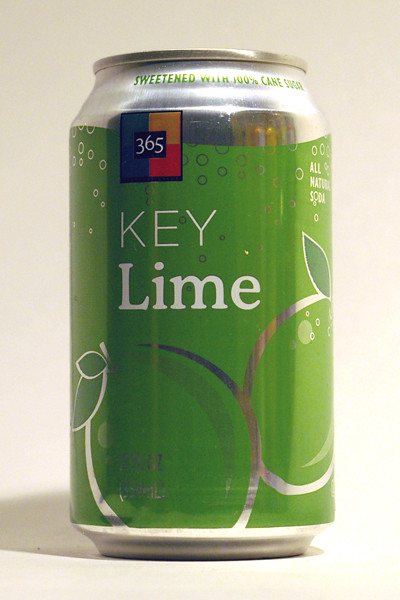A close-up, eye-level view of a soda can. The majority of the can is silver with a vivid green band encircling the middle. On this green section, there are two etched images of limes: the one on the left angled to the left, and the one on the right angled to the right. Centered on the can in white letters, it reads "Key Lime," with the word "Lime" bolded for emphasis. At the top left of the can, there is a square with a black background, featuring four small colored triangles—blue, yellow, purple, and red—in each corner. In the center of this square, the number “365” is written in white.